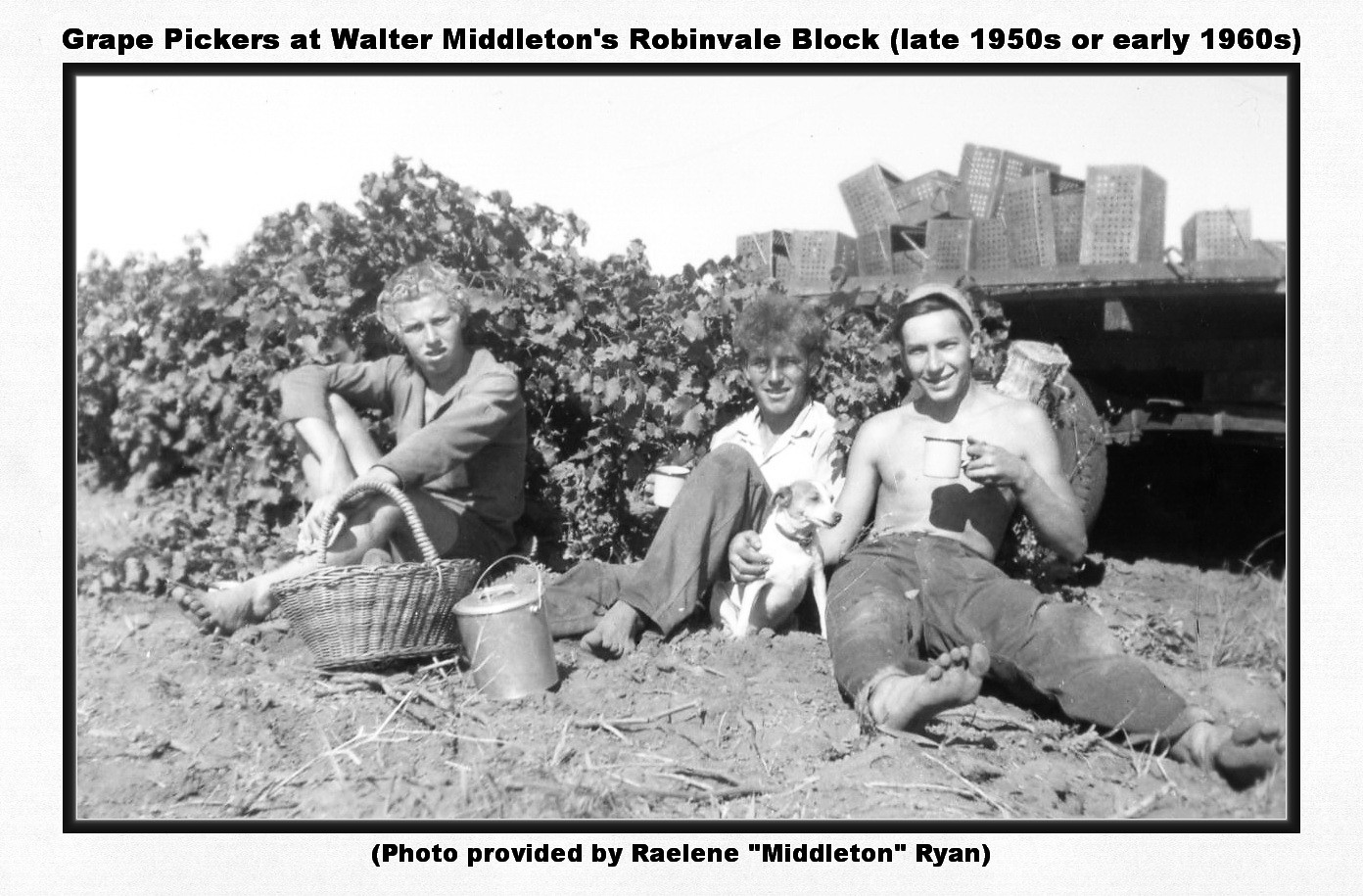This is a horizontally-oriented black-and-white photograph of three teenage boys reclining on the bare ground, framed by light gray or off-white borders. A caption at the top reads, "Great Pickers at Walter Middleton's Robin Vale Block, late 1950s or early 1960s," and at the bottom, it states, "Photo provided by Rainey Middleton Ryan." The boys are dressed in worn-out clothes: the one on the right is smiling and holding a coffee cup with an arm around a small white dog, the middle boy is wearing a white shirt and pants, and the boy on the left is dressed in clothes that seem too small for him, including tiny shorts and a shirt. None of them are wearing shoes. In front of them, there is a wicker basket, suggesting a connection to grape picking. Behind them, low shrubbery, grapevines, and what appears to be a trailer with metal containers are visible, along with stacks of collection baskets in the upper right corner, indicating their work environment.